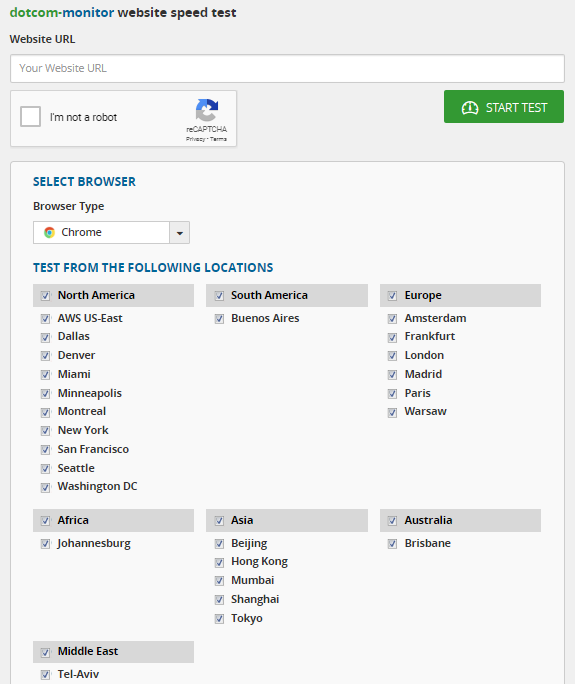This image showcases a webpage interface for an app, specifically the Dotcom-Monitor Website Speed Test. The title "Dotcom-Monitor Website Speed Test" features prominently at the upper left corner, with "DOTCOM" written in green, "Monitor" in blue, and "Website Speed Test" in black. The overall background of the page is grey.

At the bottom of the page, there's an input field labeled "Website URL" where users can enter the URL of the website they want to test. Adjacent to this is a reCAPTCHA verification system with a checkbox labeled "I'm not a robot." On the right side, there's a green button labeled "Start Test."

Below the reCAPTCHA system, the user can see a section labeled "Select Browser" in blue, with "Browser Type: Chrome" displayed next to a drop-down menu where users can choose their preferred browser. Another section below this, with text in blue, is titled "Test from the following locations," and it lists multiple geographic locations in black text where website speed tests can be conducted. These locations include:

- North America: AWS-US East, Dallas, Denver, Miami, Minneapolis, Montreal, New York, San Francisco, Seattle, Washington.
- Africa: Johannesburg.
- South America: Buenos Aires.
- Europe: Amsterdam, Frankfurt, London, Madrid, Paris, Warsaw.
- Australia: Brisbane.
- Asia: Beijing, Hong Kong, Mumbai, Shanghai, Tokyo.
- Middle East: Tel Aviv.

Many of these locations are pre-selected, highlighted in grey, indicating that their tests are activated by default.